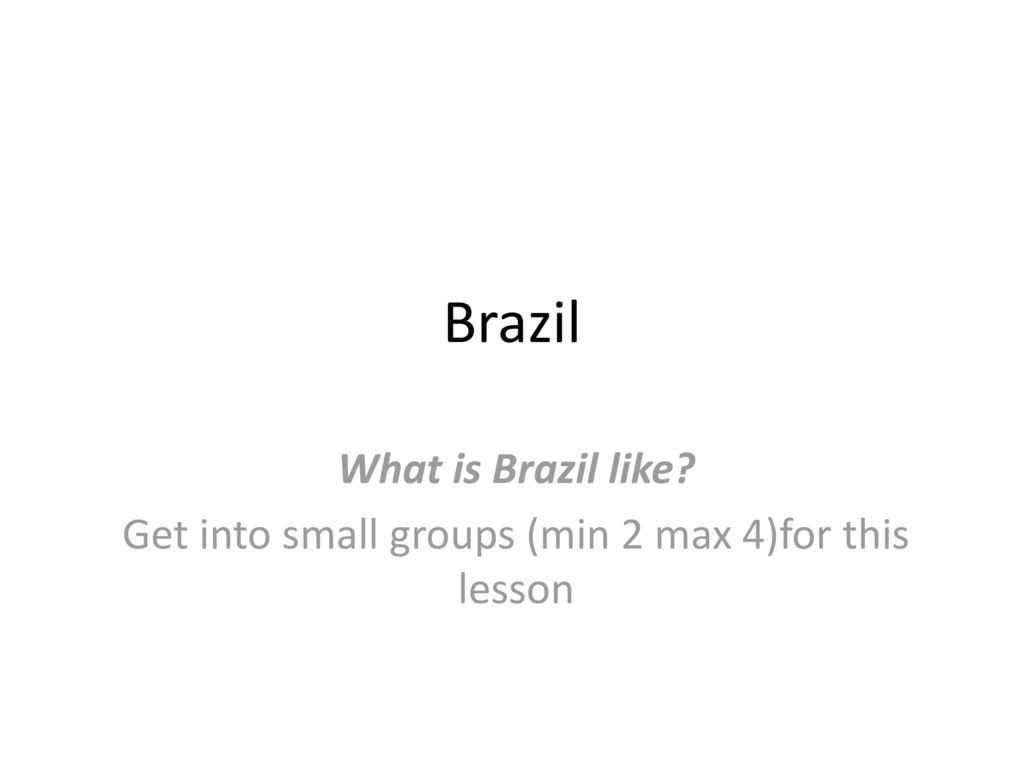The image features a predominantly white background with minimal design elements focused in the center. At the top center, the word "Brazil" is prominently displayed in bold, black capital and lowercase letters ("B" capitalized and "razil" in lowercase). Below "Brazil," there is a question in a gray font: "What is Brazil like?" with a question mark at the end.

Further down, there is an instruction in gray font that reads: "Get into small groups." This sentence is followed by a phrase in parentheses, which states: "(min 2 to max 4 minutes for this lesson)." The instructions are centered on the white background, making the phrase in parentheses extend slightly longer than the initial sentence. The word "lesson" appears at the bottom, also in gray font, and is similarly centered. There is no punctuation following the word "lesson."